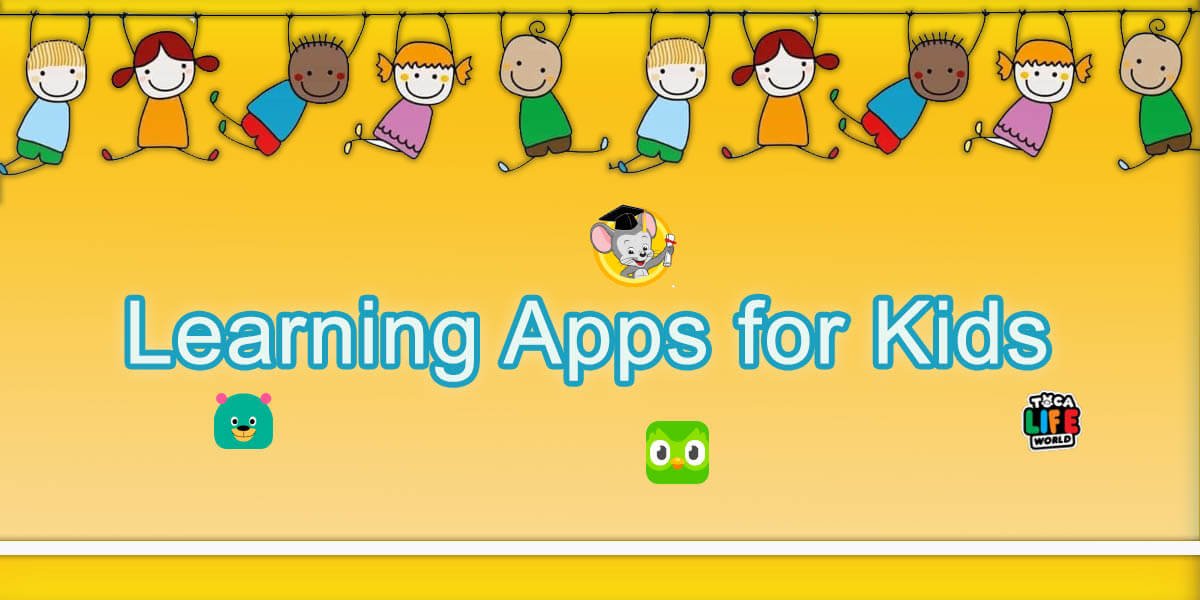This image features a vibrant website display tailored for a platform dedicated to educational apps for children. The background transitions from a beige hue at the bottom to a more vivid yellow as it ascends, with the yellow becoming increasingly pronounced towards the top. At the very top of the image, a thin horizontal black bar spans across, from which ten animated children of varying skin tones and colorful outfits are suspended, adding a lively and engaging touch to the design.

Prominently placed in the center of the image is a large yellow circle featuring a mouse icon colored in white and gray, adorned with a black graduation cap, symbolizing learning and education. Beneath this icon, the text "Learning Apps for Kids" is boldly presented in white letters with a blue outline, making it easily readable against the vibrant background.

Additionally, the left side of the image includes a cute animation of a bear, and in the middle, there is an animation highlighting the face of a bird, both characters contributing to the playful and child-friendly aesthetic of the site. On the right side of the image, the label "TCA Life World" is visible, possibly indicating the name or tagline of the educational platform. The overall design is colorful, engaging, and inviting, perfectly suited for its young audience.